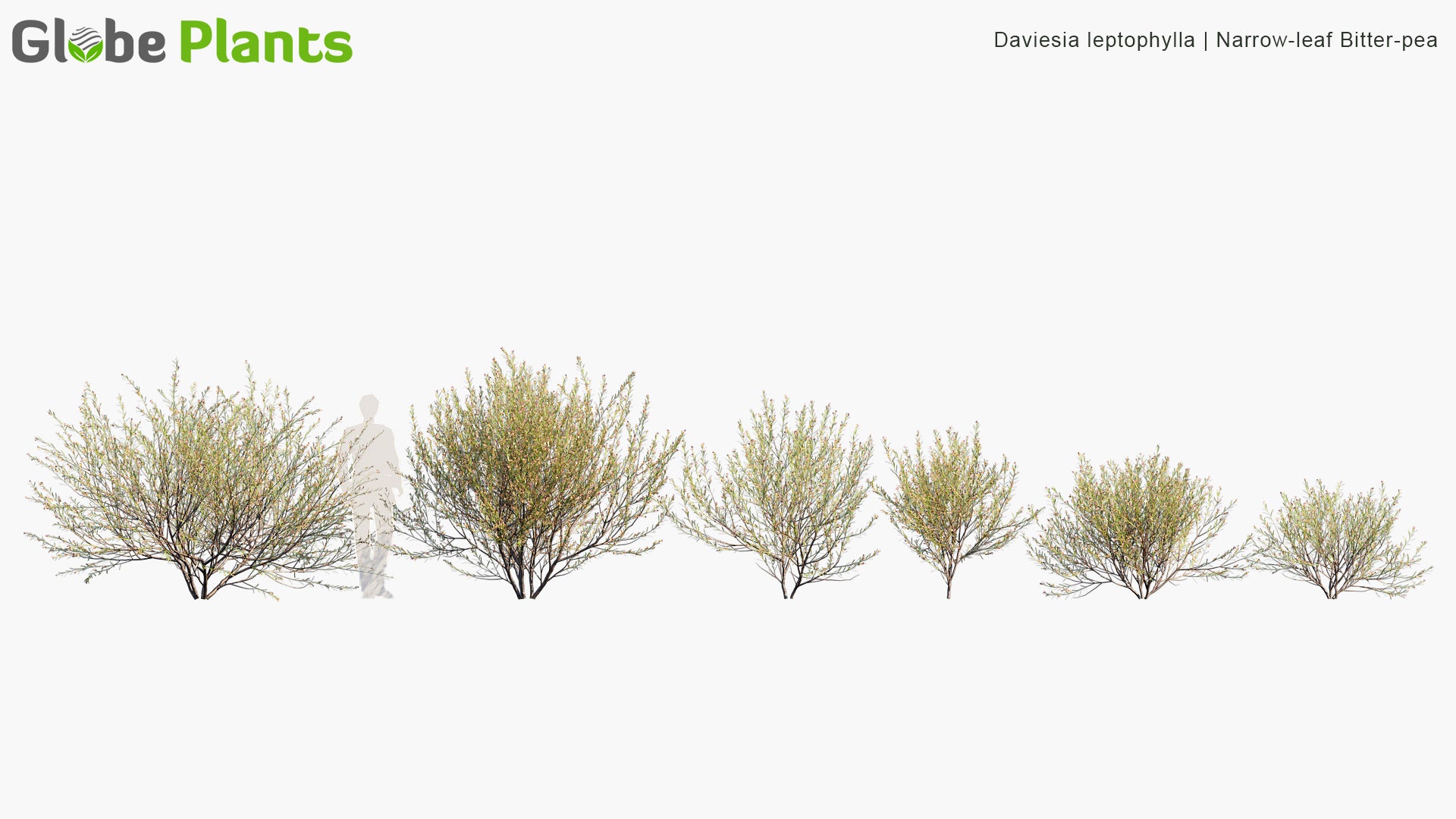This image, titled "Globe Plants," showcases the plant species Devicea leptophylla, also known as narrowleaf bitter pea. The title "Globe Plants" is prominently displayed with the word "Globe" in gray and "Plants" in green, featuring a circular "O" with green leaves at the bottom.

The image displays six variations of the narrowleaf bitter pea, arranged from the largest on the left to the smallest on the right. On the far left, a silhouette of a human being is included for scale, indicating that the largest plants are slightly taller than an average human. The variations become progressively smaller, with the smallest plants reaching about waist height.

These bushes have long, dark, thin branches that appear mostly bare, adorned with tan-colored buds or small flowers resembling the hue of a wheat field. The plants exhibit a mix of green, beige, brown, and gray tones, giving them a dried-up, bush-like appearance. The overall layout emphasizes the size gradation and distinct coloration, offering a detailed representation of this plant species.